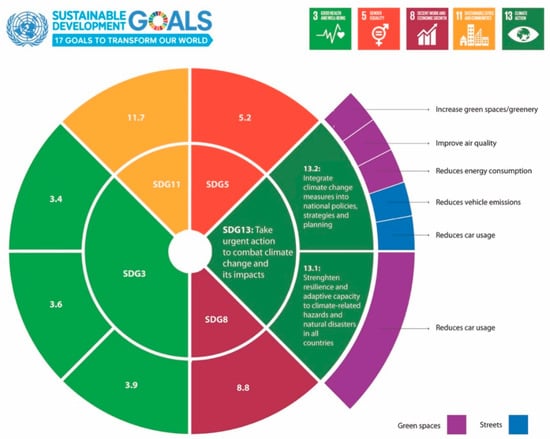This image displays a diagram illustrating the Sustainable Development Goals (SDGs), accompanied by the headline "17 goals to transform our world" in the upper left. The upper right features a blue world logo. Central to the diagram is a multi-colored circular chart or wheel, segmented into various colored sections including green, orange, red, yellow, and a darker crimson. Each segment is associated with specific logos, such as a heartbeat monitor, a gender symbol, and a stock graph, indicating different focus areas. Adjacent to this wheel are five color-coded boxes in green, orange, burgundy, yellow, and darker green, each containing relevant icons. The bottom right includes a color code where a purple square denotes green spaces and a blue square represents streets. The diagram explicitly links these visual elements to goals like increasing green spaces, improving air quality, reducing energy consumption, and cutting down vehicle emissions.